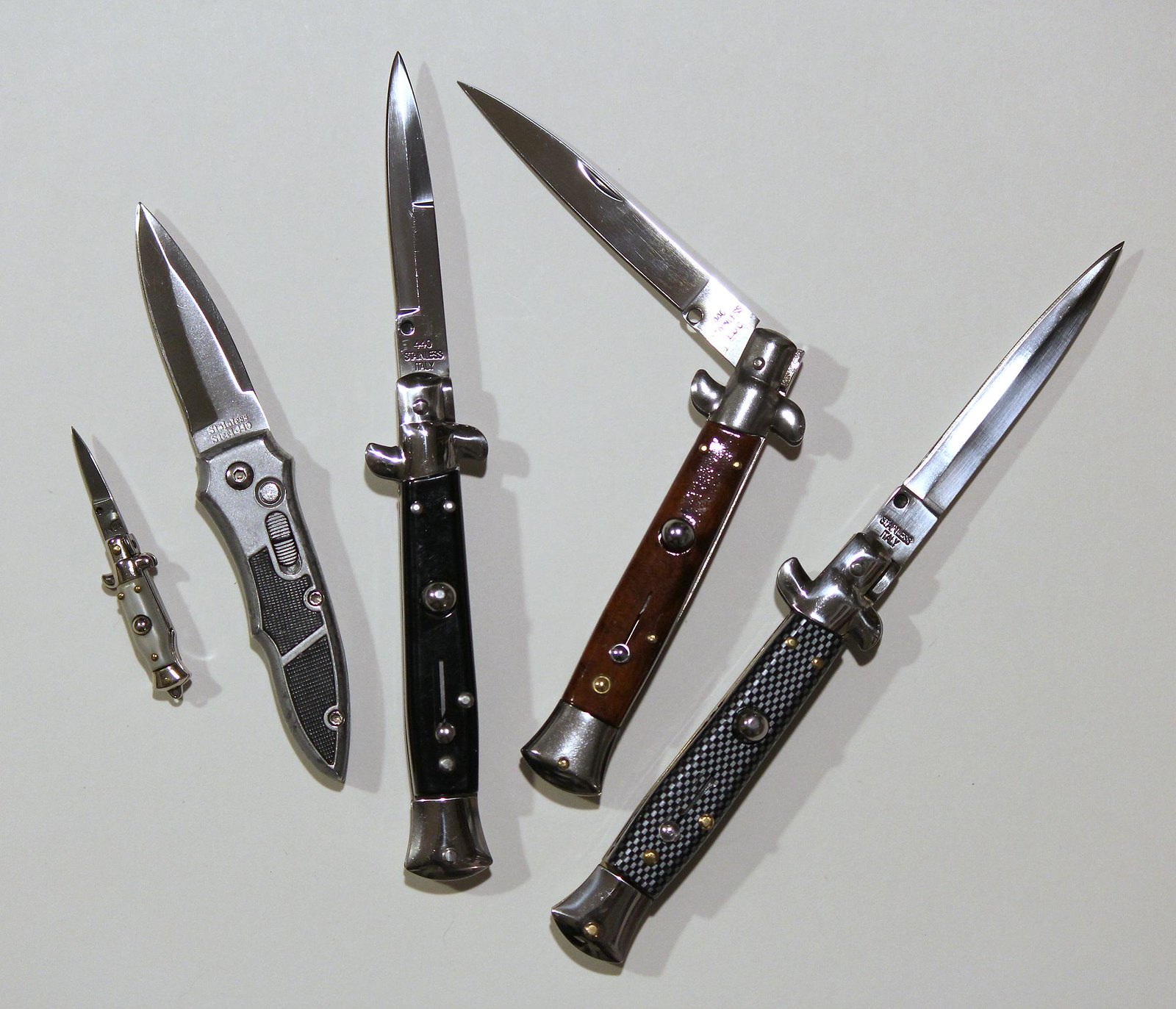The photograph showcases a collection of five diverse switchblades meticulously arranged on a white surface, casting pronounced shadows from the upper right to the lower left. Each knife is pointed upward, demonstrating a variety of handle designs and blade lengths. 

The first knife on the left is a very small pocket-sized switchblade with an ornate handle featuring a round button, and a blade likely no more than an inch long. The second knife appears to be a foldable pocket knife with knurling on the handle and a blade approximately a couple of inches long. 

The third switchblade stands out with a black handle accented by a decorative S-scroll pattern and metal caps at both ends. Its blade is about two and a half inches long. The fourth switchblade, notable for its inlaid wooden handle and metal caps, has a blade positioned at a near-perpendicular angle to the handle, suggesting it is around three and a half inches long. 

Lastly, the fifth knife sports a carbon fiber-like handle with metal caps and a slender blade, bearing a stamp indicating it was made in Italy. This blade is roughly three and a half inches long, situated on a slightly longer body. 

Together, these knives exemplify a range of sizes and designs, set against a stark background, highlighting their intricate details and shadow play.